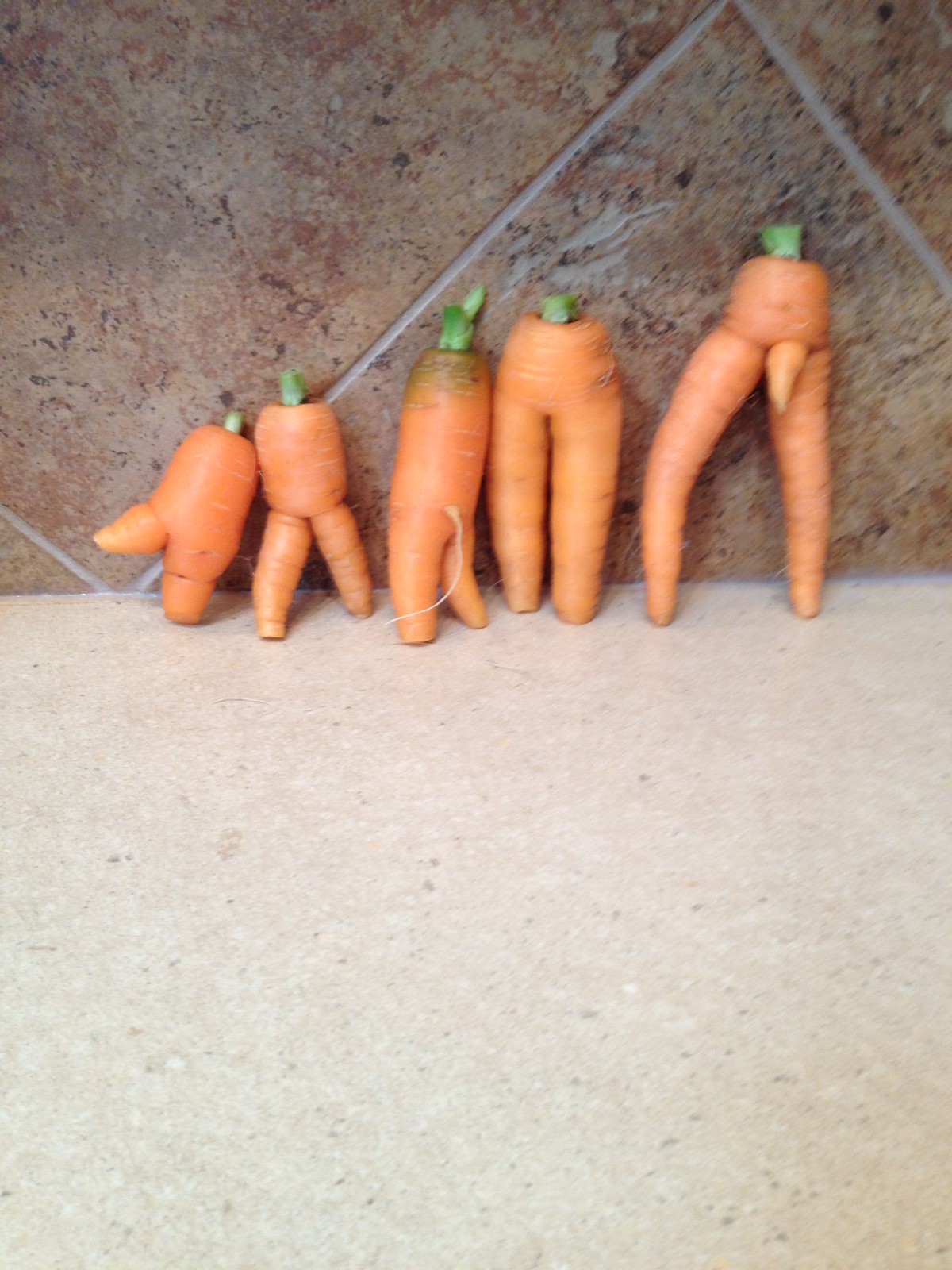This photograph captures a whimsical arrangement of five misshapen carrots, each resembling human legs, set against a light brown corian countertop and a backdrop of brownish tiles with white grout lines. The backdrop creates an illusion that the carrots are standing on a light grayish brown cement floor, dancing against the wall. 

From left to right, the carrots are arranged from the shortest to the tallest. The shortest carrot on the far left is squat and stubby, sporting a green stem on top. It has two short legs, one kicking out to the side while the other remains grounded. The next carrot is slightly taller with a stout body and a pair of legs spread out just enough to maintain balance, although, like the others, it leans against the wall for support. The middle carrot features a green stem and two legs, with a small root protruding from the back, appearing as a tail. This carrot seems to stand almost upright. The penultimate carrot is slightly taller and has a more defined, uniform shape, almost like it’s wearing “mom jeans,” and also showcases two legs. The tallest carrot on the far right strikes a dramatic pose with one leg straight and the other bent as if it's mid-dance, featuring a green stem and a small nub between its legs, adding to its character.

All the carrots share a vibrant orange color and a playful appearance, creating a charming and humorous tableau.